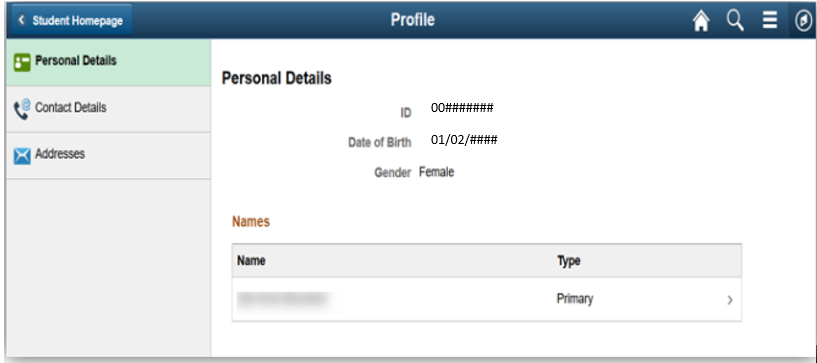In the student homepage profile image, the top section features a blue, almost grayish-blue rectangular banner with a smaller white rectangular button overlaid. This button, positioned towards the left, is labeled "Student Home Page." Moving to the center of the image, the word "Profile" is displayed prominently in white print. To the right of this, several icons are visible: a house icon representing the homepage, a magnifying glass for search, an icon with three horizontal lines possibly for a menu, and a circular icon in the corner.

Below this, the section titled "Personal Details" is highlighted in green, indicating it has been selected. Accompanying this header is a darker green icon next to it. Further down, there are additional sections such as "Contact Details" accompanied by a phone icon, and an "Addresses" section indicated by an envelope icon in blue.

In the "Personal Details" section, the student’s information includes fields for ID, date of birth, gender – marked as female, and names, though the specific details of their names are blurred out for privacy.